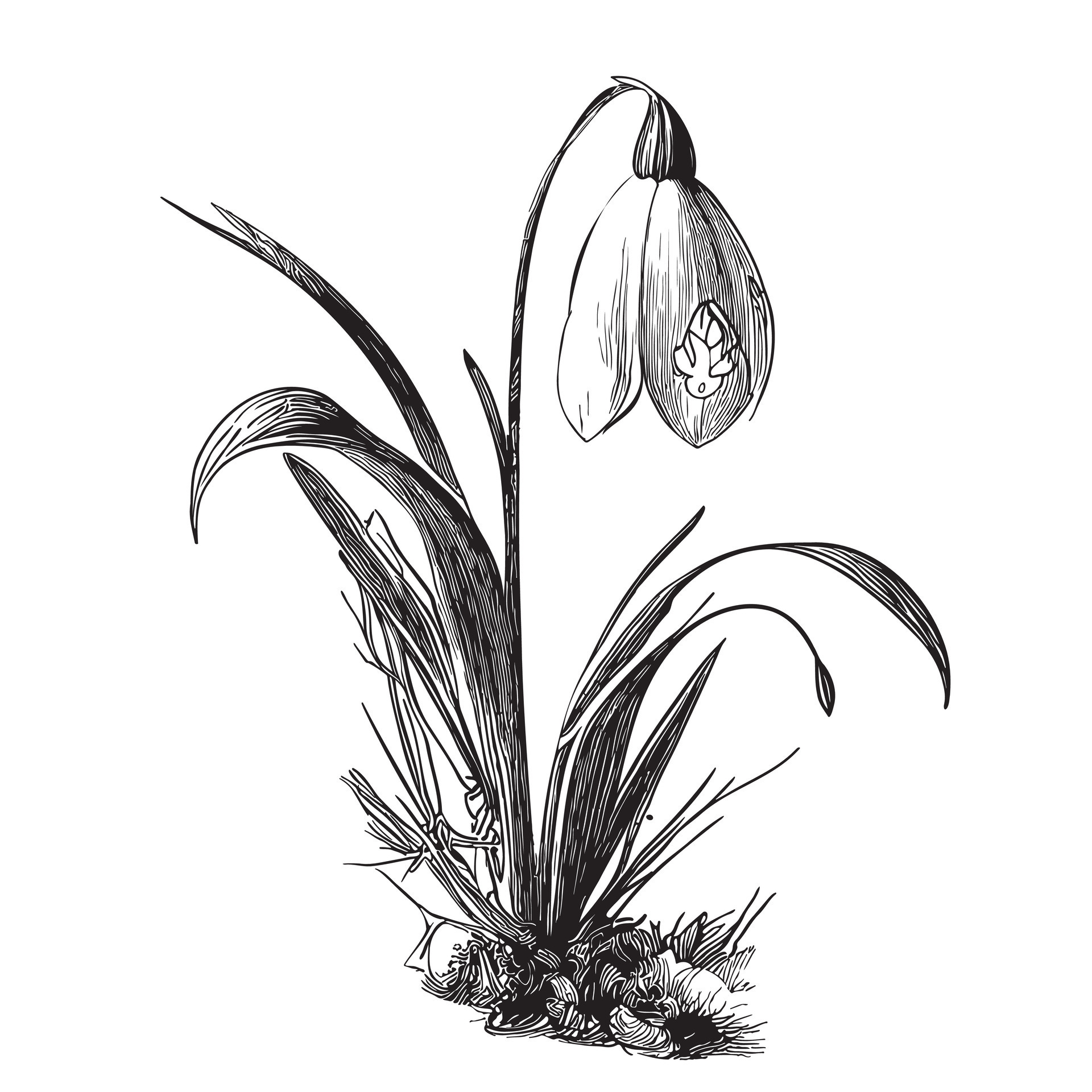The image is a detailed black and white sketch of a flowering plant, most likely a lily or tulip, with a distinctive, upside-down bloom that hangs downward, resembling a lamp. The petals are white with textured black lines, creating a contrast that highlights their delicate structure. Thick, curved leaves extend in C shapes from the stem, looping outwards in various directions, suggesting a sense of drooping or wilting. At the base of the plant, there are additional smaller leaves or blades of grass, along with a suggestion of rocky ground. The background is stark white, drawing the viewer’s focus entirely on the intricately designed flower and its detailing, including what appears to be either an etched design or a small spider-like figure on one of the petals.